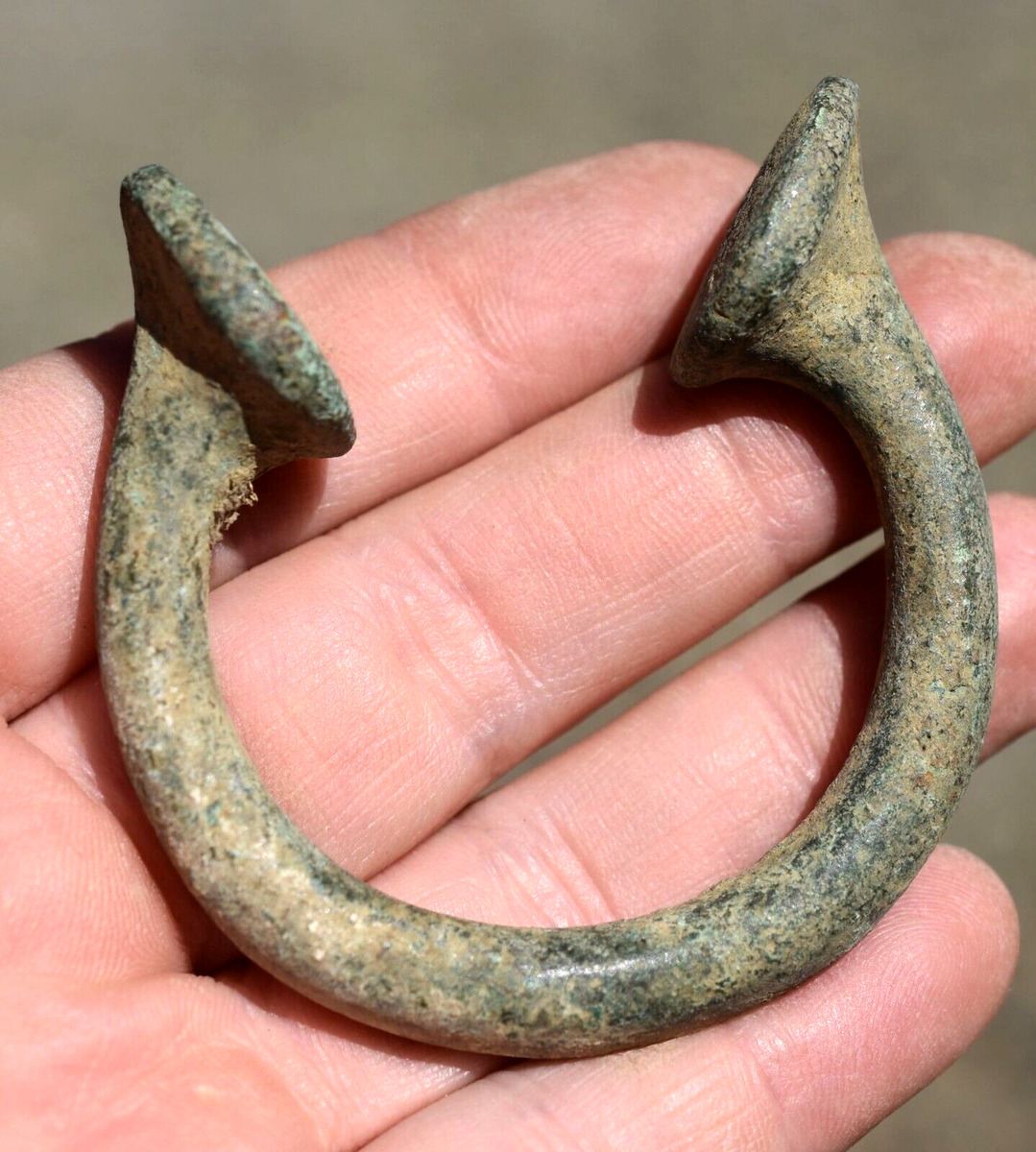This close-up image, in portrait orientation, features the weathered hand of a Caucasian man extending from the lower left corner, with the fingers holding a small, U-shaped horseshoe that points toward the upper right. The fingers grip the horseshoe tightly, revealing the hand's rough, work-worn texture. The horseshoe, composed of aged and tarnished metal, exhibits a predominantly gray tone interspersed with light gray, dark gray, white, tan, and beige discoloration and pitting, indicating significant wear and age. The incomplete ring of the horseshoe, possibly made of steel, broadens near the opening, ending in a smoothed, rounded edge. The background of the image is a slightly mottled grayish-brown, devoid of any distinct features, further emphasizing the detailed focus on the hand and the antique horseshoe.